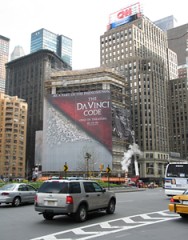The photo depicts a bustling urban scene, likely Atlanta, given the prominent tall building displaying the CNN logo – indicative of CNN's headquarters. Beside this structure, a smaller building showcases a massive advertisement for "The Da Vinci Code" movie, identifiable by its text and red and gray design elements, evoking an early to mid-2000s vibe. The scene is captured at street level, featuring various vehicles including a bus, a taxi, and a boxy SUV characteristic of that era. Below the advertisement, people can be seen walking and milling about, contributing to the city's vibrant morning atmosphere. The sky appears cloudy, casting a diffuse light over the scene, with some steam or smoke rising nearby, adding to the dynamic urban setting.